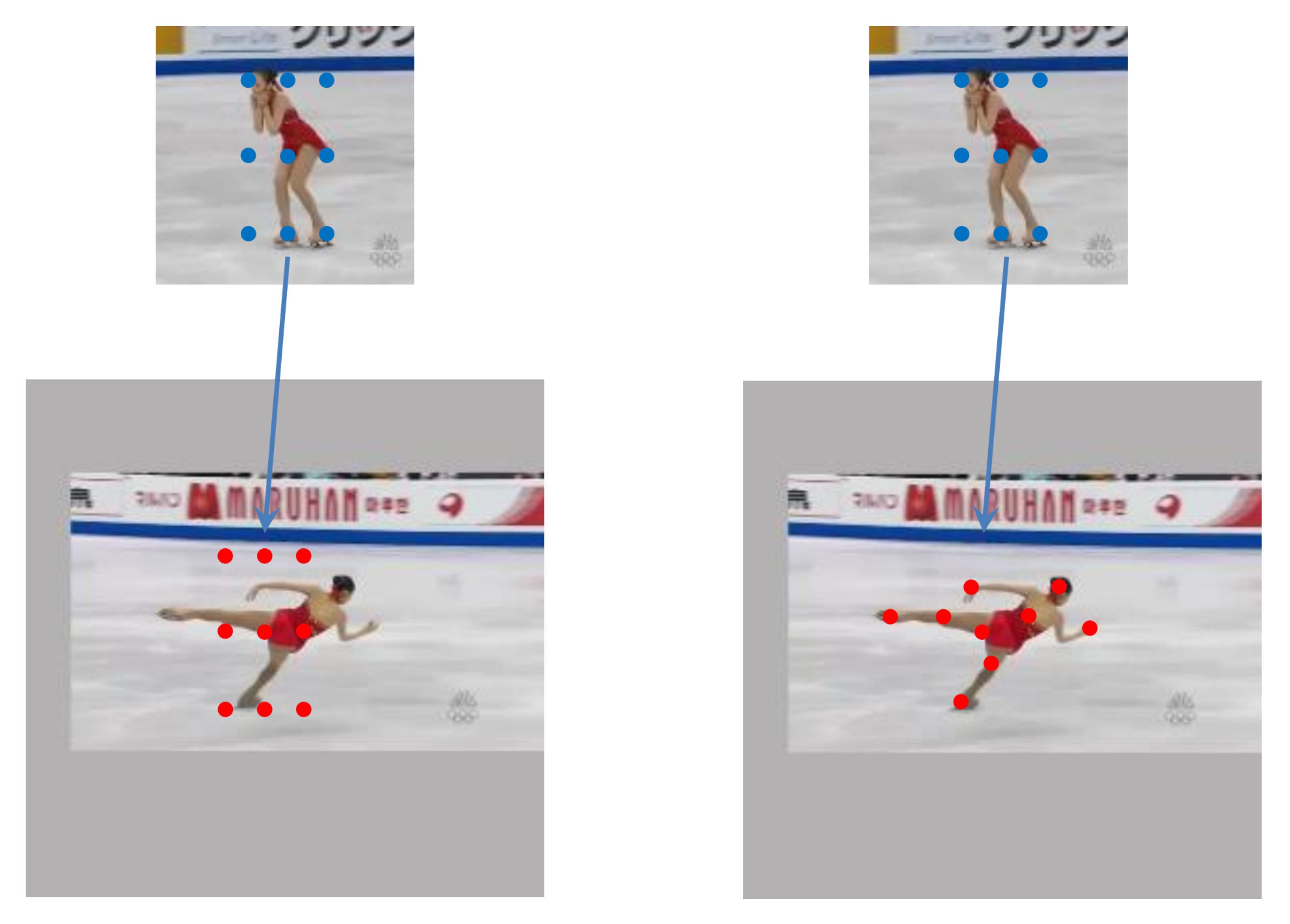This series of four photographs depicts an ice skater in various poses on an ice rink, with each image annotated with colored dots and arrows. The skater, wearing a red dress, is shown in two smaller images at the top and two larger images at the bottom. In the top two images, she is leaning forward with her head in her hands, and a grid of blue dots is superimposed over her. A blue arrow connects these images to a larger image below, where the skater is captured in a different position—her leg outstretched as if preparing to spin. The grid of dots transitions from blue to red, now detailing specific points of articulation: three on each leg, one on the torso, one on each arm, and one on the head. A Japanese advertisement with the word “Maruhan” is visible in the background, indicating the location is in Japan. Each photograph also bears the Olympic logo in the bottom right corner, suggesting the context of an Olympic event.